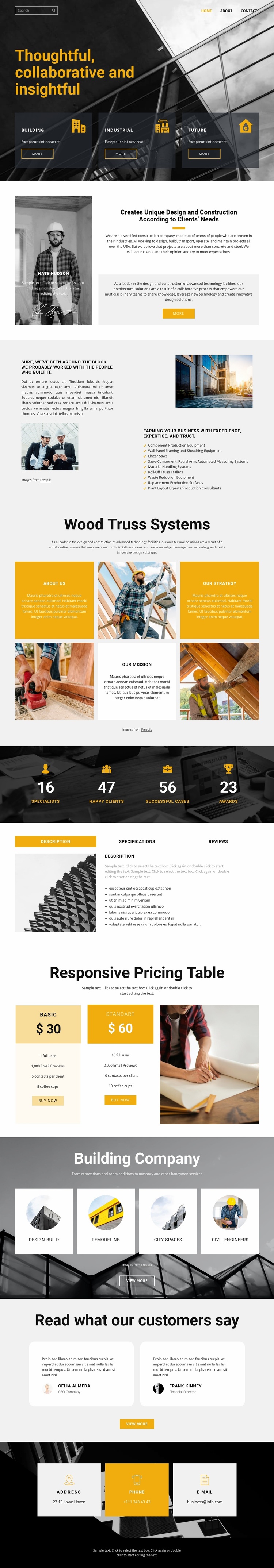The image depicts a detailed layout of a web page designed in a vertical rectangular format. At the very top, there's a thin horizontal bar that spans the entire width of the image, featuring the caption: "Thoughtful, collaborative, and insightful." Below this bar, a staircase railing is visible.

Following this, the main content begins with an image of a man wearing a hard hat, giving the appearance of a construction worker. To the right of this image is text, though it is too small to be legible. Moving further down the page, there is another text box accompanied by an image of two workers consulting over a paper document. Adjacent to this is an outdoor shot, possibly of a factory, with accompanying small print text.

The next title reads "Wood Truss Systems," introducing a section composed of six smaller rectangles, arranged in two rows of three. Below this section is a black rectangle featuring an icon with numerical data underneath.

Continuing down, there is another section with two rectangles: one displaying an image that appears to be of rope, and to the right, some printed text. Following this is a "Responsive Pricing Table," represented by a row of three blocks.

Towards the bottom of the page is a gray rectangle that reads "Building Company," which includes four small blocks. This is followed by a section titled "Read What Our Customers Say," featuring two blocks of customer testimonials.

The page concludes with a black rectangle containing three information boxes: one white, one orange, and another white, closing out the web page's design.